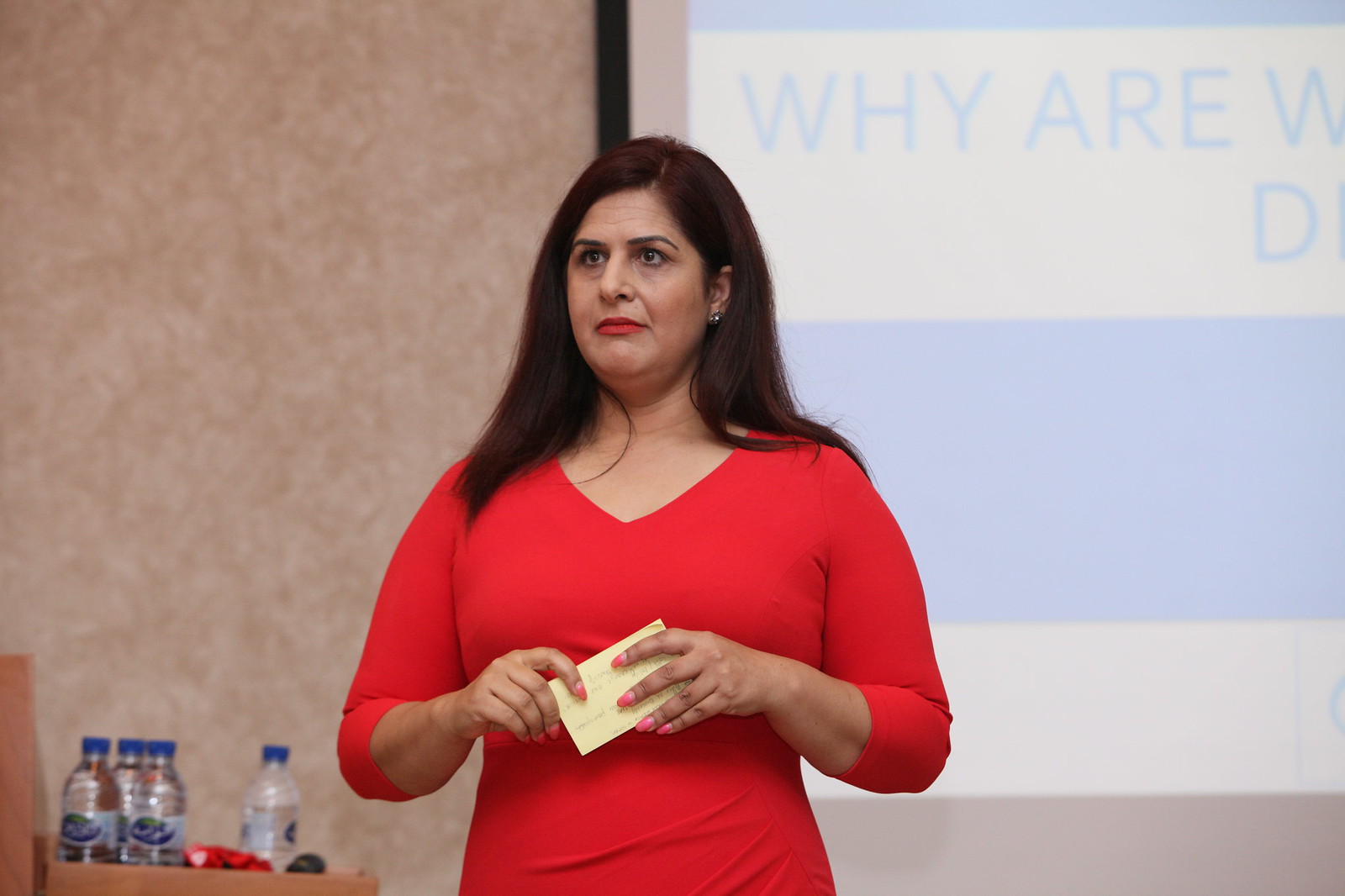The image is a color photograph taken indoors in landscape orientation, depicting a middle-aged woman at the center, seen from the waist up. The woman, who has straight, shoulder-length brown hair parted on the side and tucked behind her left ear, is facing slightly to the left and gazing off in that direction. She has lighter skin with subtle signs of aging, including a slight droop to her face and a hint of a double chin. Her makeup includes bright reddish-orange lipstick, and she is wearing a reddish-orange 3-quarter sleeve top with a V-neck. Her arms are bent at the elbows, and she holds a yellow 3 by 5 card with pink-painted fingernails.

In the background on the left side, a brown mottled wall occupies the lower corner beside a table that holds four bottles of water. On the right side of the image, a projector screen features light blue and white horizontal stripes, partially showing the letters "YRW" and "D" below them. The setting suggests an indoor seminar or presentation, implied by the woman's contemplative or possibly disturbed expression and the arrangement of objects around her.